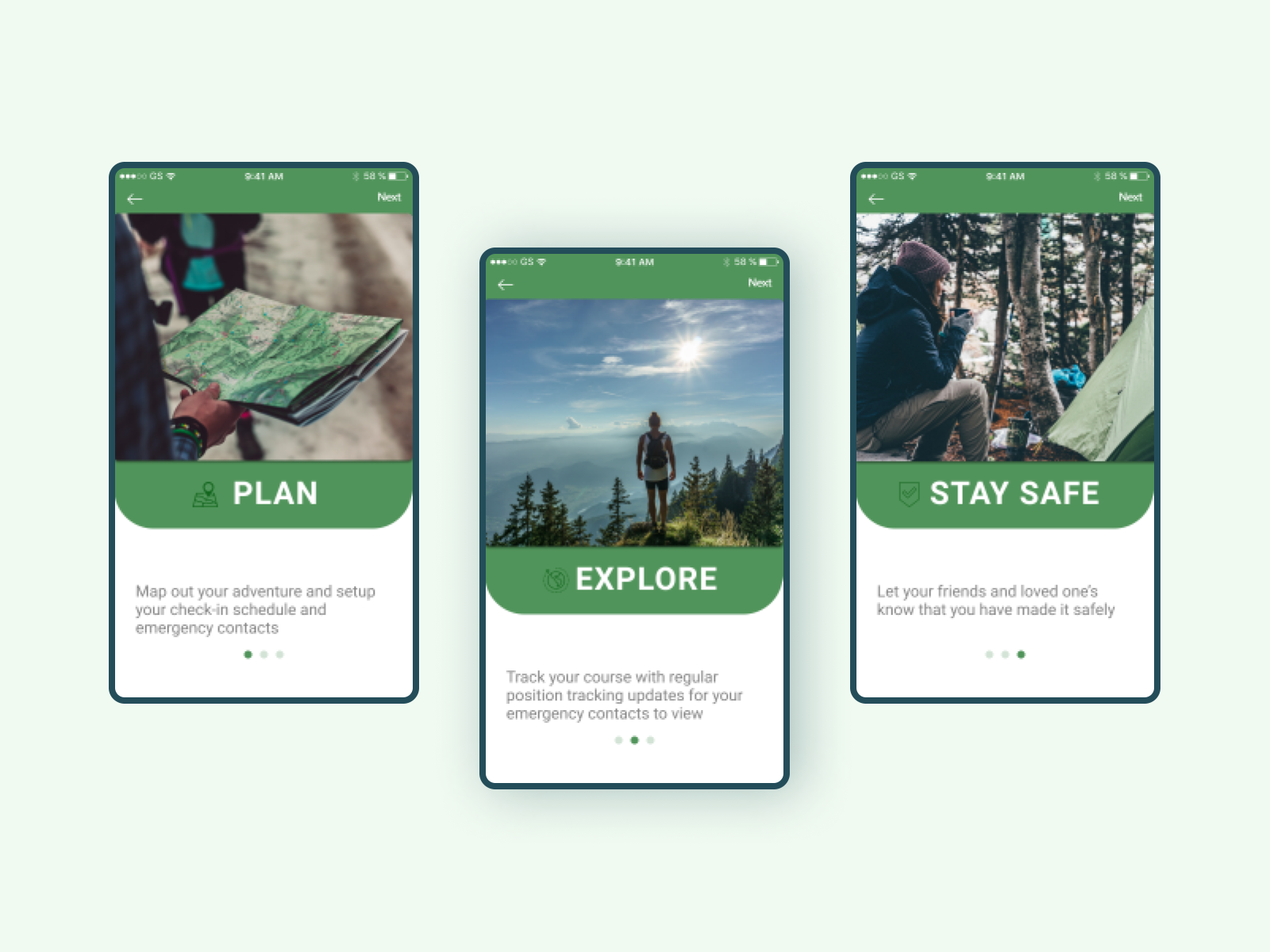The image features a light gray background and displays three smartphones positioned side by side from left to right, each showing the same website. The webpage is characterized by a dark green stripe at the top.

- The smartphone on the left showcases an image of a person holding a map. Beneath this, a green box contains the word "Plan" in bold letters. Below this box, there is a white outline with the text: "Map out your adventure, set up your check-in schedule, and emergency contact."

- The middle smartphone presents a green background with several phone icons at the top. Below these icons, there's an image of a man standing atop a mountain, surrounded by trees, gazing into the vast distance. Under the image, the word "Explore" is prominently displayed, followed by: "Track your course with regular position updates for your emergency contacts."

- The smartphone on the right depicts an individual camping in the woods. Directly below the image, the text reads: "Stay Safe." Further down, it elaborates with: "Let your friends and loved ones know that you have made it safely," accompanied by three dots underneath.

This detailed setup highlights different aspects of the website's features, focusing on planning, exploring, and ensuring safety during adventures.